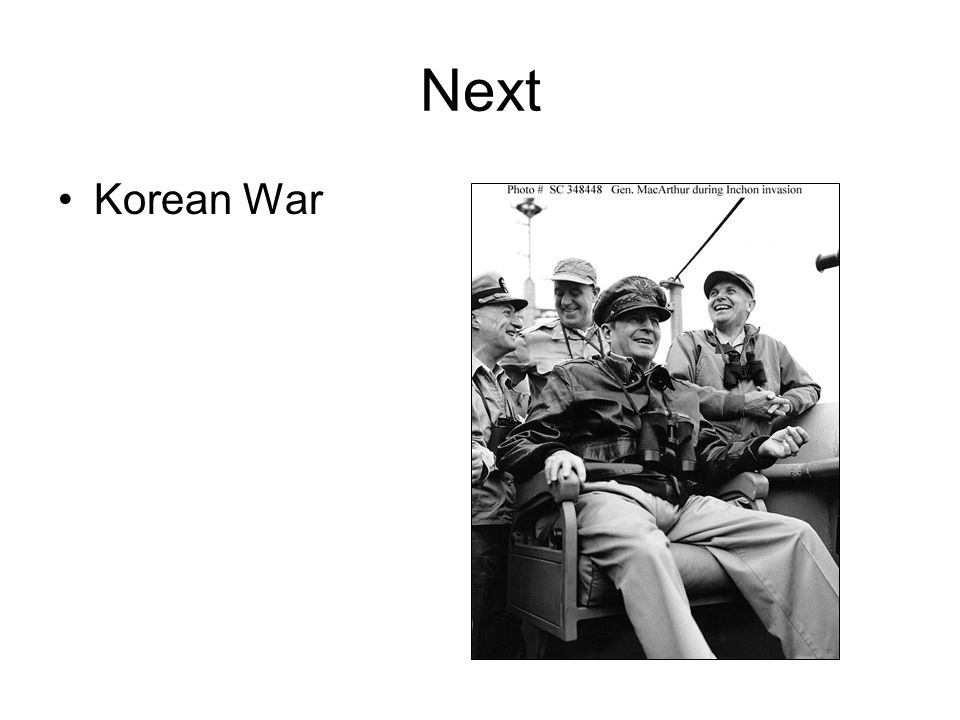This black and white photograph, titled "Korean War," depicts a scene from the Inchon invasion. It features four middle-aged to older men, likely in their 50s or 60s, all wearing military uniforms and hats. The man in the front, seated in a captain's chair, is identifiable by his leather jacket, black cap, and a pair of binoculars dangling from his neck. The three men standing behind him, all of whom are smiling, wear lighter cotton jackets. The background appears to be the sky, and elements such as ship pillars and cables are visible, indicating that they are on the deck of a naval ship. Above the image, a bold black text reads "NEXT," while to its left, a bullet point marked "Korean War" is prominent. Additionally, the photo is framed with a thin black border, and beneath it, the caption "General MacArthur during Inchon invasion" is noted, alongside the photo number SC-348-448.